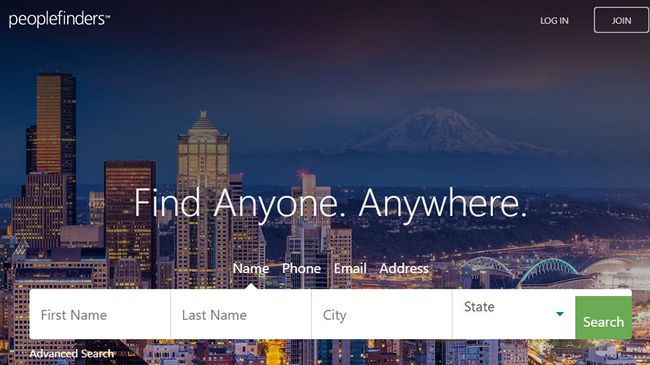Screenshot Description:

The screenshot is in landscape mode and depicts a vibrant, bustling cityscape as the central background. Beyond the city, a serene body of water stretches out, leading up to a majestic, snow-covered mountain that towers in the distance, creating a picturesque, layered backdrop. 

In the upper left-hand corner of the image, the "People Finders" logo is prominently displayed. This logo represents a website designed to help users search for individuals by name and state location, pulling up relevant information.

On the upper right-hand corner, there are two distinct buttons: one for "Login" and a white-bordered button labeled "Join."

Centrally positioned on the screenshot is the bold tagline "Find anyone. Anywhere." Beneath this text, there are four navigational tabs labeled "Name," "Phone," "Email," and "Address."

Directly under the "Name" tab, a form appears allowing users to input details such as first name, last name, city, and state, with the state selection available via a drop-down menu. To the right of this form, a noticeable green "Search" button invites users to execute their query.

In the bottom left-hand corner of the screenshot, a link marked "Advanced Search" is available, providing an option for more detailed search parameters.